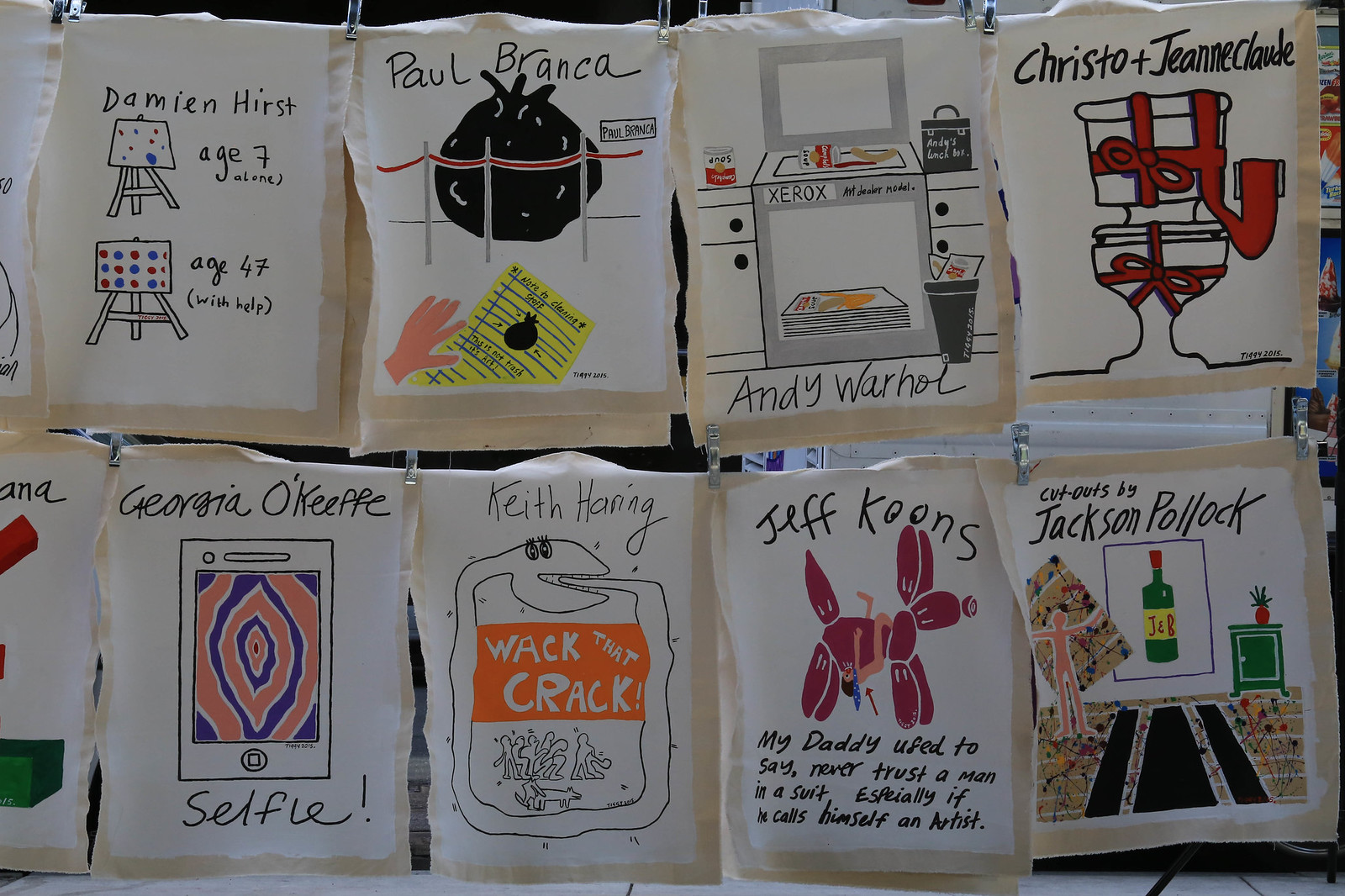The image showcases eight pieces of art hanging on a clothesline with clothespins, resembling a line of drying clothes or bags. Each piece humorously references a different famous artist, blending words and drawings in a playful manner. Starting from the top left, the first artwork features two easels with dots, referencing Damien Hirst: one drawing labeled ‘age 7’ and the other ‘age 47 with help’. Next is a piece labeled ‘Paul Branca’ featuring a hand holding a sticky note with a strawberry behind bars. The third artwork, labeled ‘Andy Warhol’, depicts a stove with the word ‘Xerox’, flanked by a Campbell's soup can and a wastebasket. The fourth piece, attributed to Christo and Jeanne Claude, shows a toilet wrapped with red ribbon.

On the bottom row, the first piece is labeled ‘Georgia O’Keeffe’ and shows colorful squiggly lines with the word ‘selfie’. Next is a piece labeled ‘Keith Haring’ with the phrase ‘whack that crack’ and a drawing of a snake eating its own tail. The following artwork, attributed to Jeff Koons, depicts a red balloon dog and an inscription that humorously mentions not trusting men in suits who call themselves artists. The final piece in the bottom row is titled ‘Jackson Pollock’ and includes images of a J&B bottle, a man holding a painting, and a green dresser with a pineapple on it. The collection cleverly integrates iconic styles and motifs of these artists into quirky, imaginative pieces.